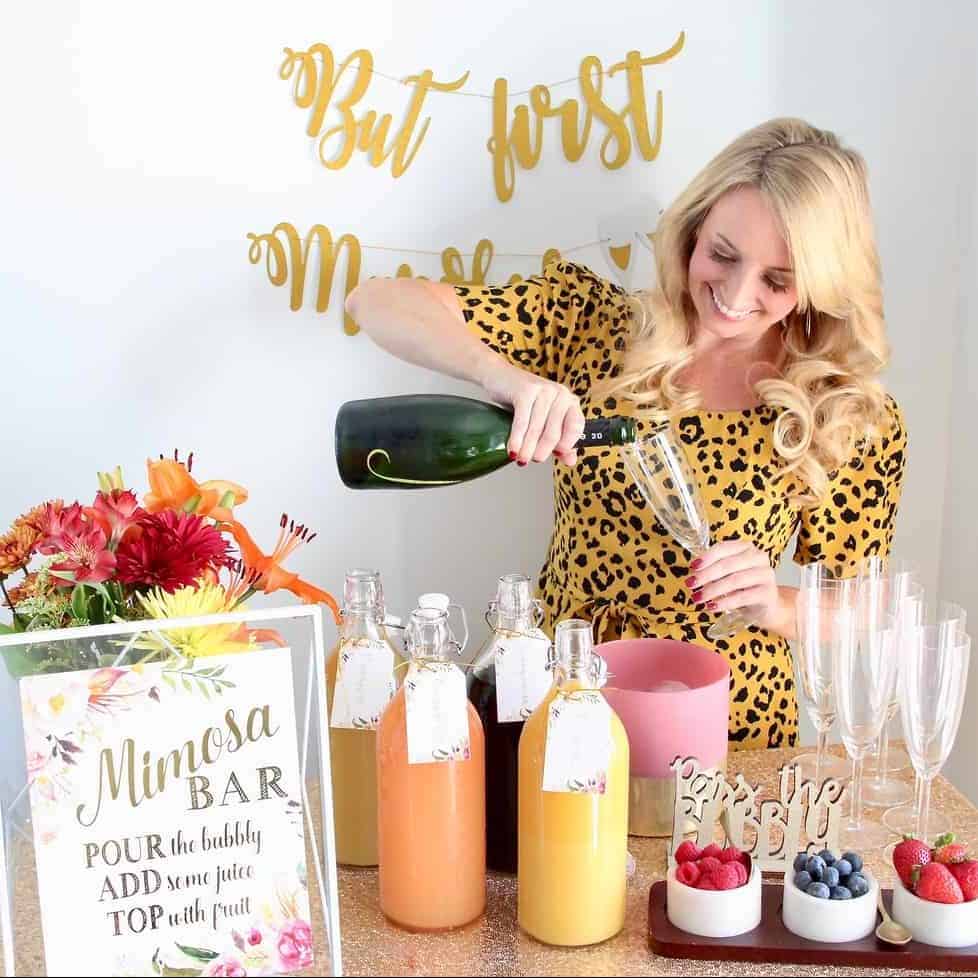In this lively celebration scene, a joyful blonde woman, dressed in a yellow leopard print outfit, is pouring champagne into a flute glass. Behind her, a partially obscured banner reads "BUT first..." against a white wall. To the lower left, a sign clearly marked "Mimosa Bar" instructs guests to "Pour the bubbly, add some juice, top with fruit." The table in front of her is adorned with a colorful array of four bottles containing dark, orange, yellow, and pale green juices. There are also plates filled with fresh berries, including blueberries, raspberries, and strawberries, along with multiple empty champagne flutes ready for use. A vibrant bouquet of flowers to the left adds to the festive décor, emphasizing the celebratory atmosphere of the setting.